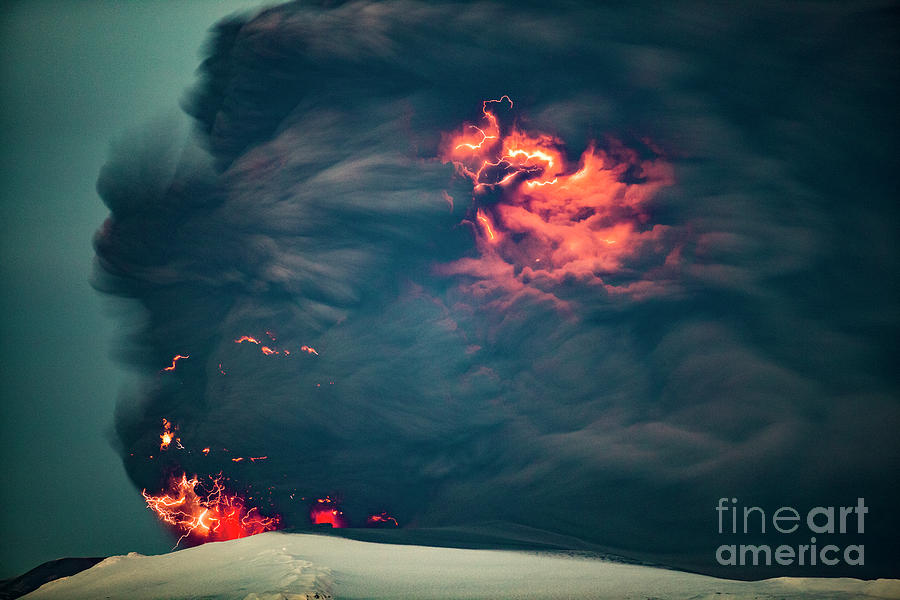This image is an evocative illustration of a wildfire in a sandy, desert-like environment. Dominated by towering plumes of dark black and gray smoke, the scene is accentuated by vivid orange and red flames flickering in both its upper and lower sections. The smoky atmosphere gives way to hints of fiery glow, sporadically illuminating the dense haze. Sparse yet strikingly bright patches of fire add a dynamic intensity to the ominous clouds. Amidst the chaos, subtle streaks of red lightning pierce through the smoky veil, adding a surreal, almost apocalyptic feel to the scene. The sky above is a murky, foggy blue, enhancing the eerie and foreboding ambiance. In the bottom right corner, the text "Fine Art America" is prominently printed in blue, identifying the source of this hauntingly compelling artwork.